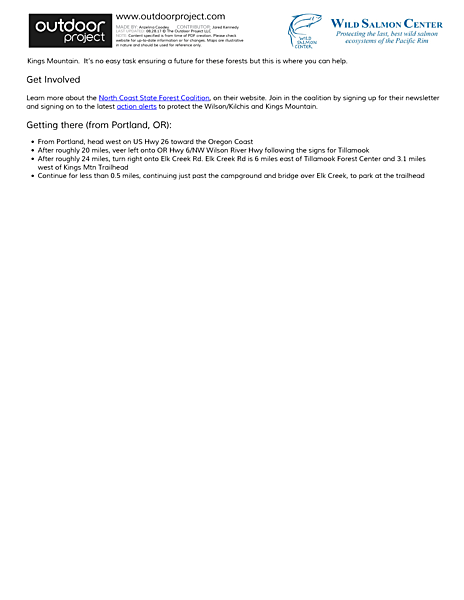The image appears to be a promotional screenshot from the website www.outdoorproject.com. On the left side of the image, there is a black box with the text "Outdoor Project" written in all lowercase letters. Below this, a block of tiny print is visible.

Moving towards the right, there's a graphical representation of a fish drawn with a blue pen, accompanied by the text "Wild Salmon Center" both above and beside the drawing. The caption "Protecting the Last Best Wild Salmon Strongholds of the Pacific Rim" underscores the overlay.

Below these elements, there is a bold headline that reads "Kings Mountain." The accompanying text highlights the challenges of ensuring the future of these forests and encourages reader involvement. Below this narrative, a prominent button labeled "Get Involved" is positioned. Further instructions prompt readers to learn more about the North Coast State Forest Coalition on their website, join the coalition by subscribing to their newsletter, and receive the latest action alerts to aid in the protection of the Wilson Kings Mountain area.

Additionally, the image includes directions to Kings Mountain from Portland, Oregon, listed as four bullet points. Notably, the terms "North Coast State Forest Coalition" and "Action Alerts" are highlighted in blue, indicating clickable links.